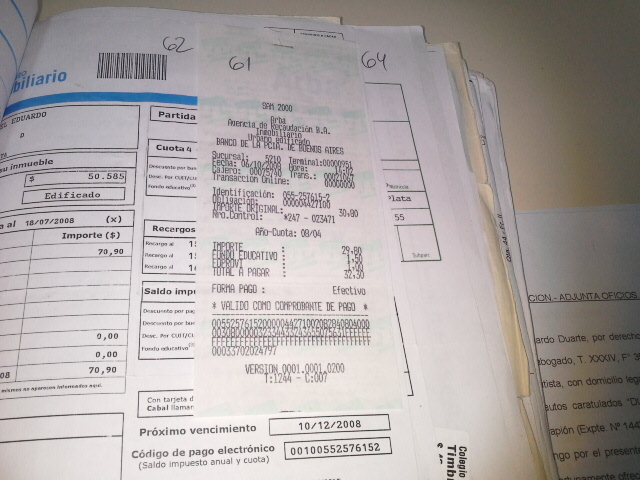This image captures a collection of documents, seemingly involved in bookkeeping or accounting, displayed on a flat, brown surface. Central to the image is an open folder, with a stack of papers spread across it. The foremost paper has a receipt stapled to its top, which indicates a total sum of $32.30. This receipt is labeled with "SAM-2000 ARBA Anarcia," suggesting it might be in a foreign language, possibly Spanish or French.

The primary document beneath the receipt features a variety of details. The number "62" is prominently marked in the center, accompanied by a barcode just underneath. Additional numerical markings, including a "61" at the top left and a "64" at the top right, are also visible. The document appears to be an invoice, as it contains elements such as a company's name at the top, a blue line, and various financial details such as import taxes. The date "10-12-2008" is printed at the bottom, reinforcing the document's age and the meticulous nature of the accounting involved.